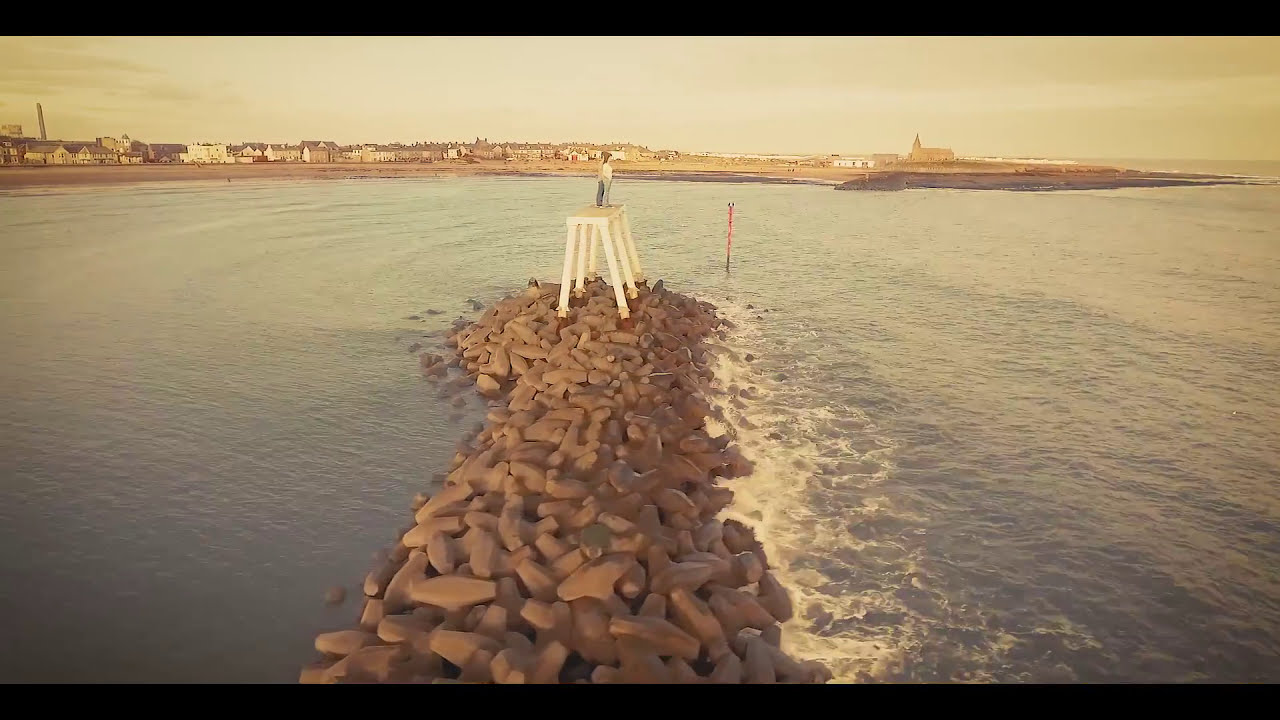The image showcases a coastal scene featuring a man-made peninsula extending into a calm, blue ocean or lake, constructed out of what appears to be piled, old metal anchors and beige rocks. At the tip of this makeshift island stands a white stool or stand with an unclear shape atop it, possibly a statue or a bird. The water appears relatively shallow, creating a jetty effect that helps protect the tranquil sandy beach from rougher waves. The shoreline is populated with numerous houses, varying in color from white to tan, many with gray rooftops. The sky has a yellow and white tint, suggesting the sun is high and bright, evoking a warm atmosphere. Notably, there is a large tan church-like building on the right side of the image, and a distinct red-and-black pole protruding from the water nearby. This idyllic coastal landscape, with its visible crashing waves and serene residential backdrop, paints a vibrant picture of a picturesque beach town.